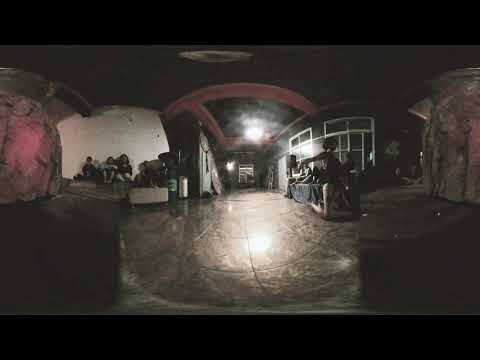In this intricate panoramic image, we observe a dimly lit underground or indoor setting characterized by walls adorned with textured faux rocks, giving the illusion of a cave-like environment. Dominating the scene are multiple seating arrangements: to the left in the mid-distance, a group of three individuals sits against the rock-like wall, while to the right, a solitary person is perched on a low table or structure. The floor, resembling rough, textured tile, enhances the rugged ambiance. As we look further into the image, there is a noticeable bright light source in the distance that reflects off various surfaces, adding depth and contrast to the predominantly dark scene. The overall color palette ranges from light red and off-white to shades of tan, brown, and deep black, contributing to the mysterious atmosphere. An arched ceiling caps the corridor stretching ahead, with cabinets or tables lining the right side. This setting, with its combination of stone-like structures and seating areas, evokes a surreal, subterranean milieu.